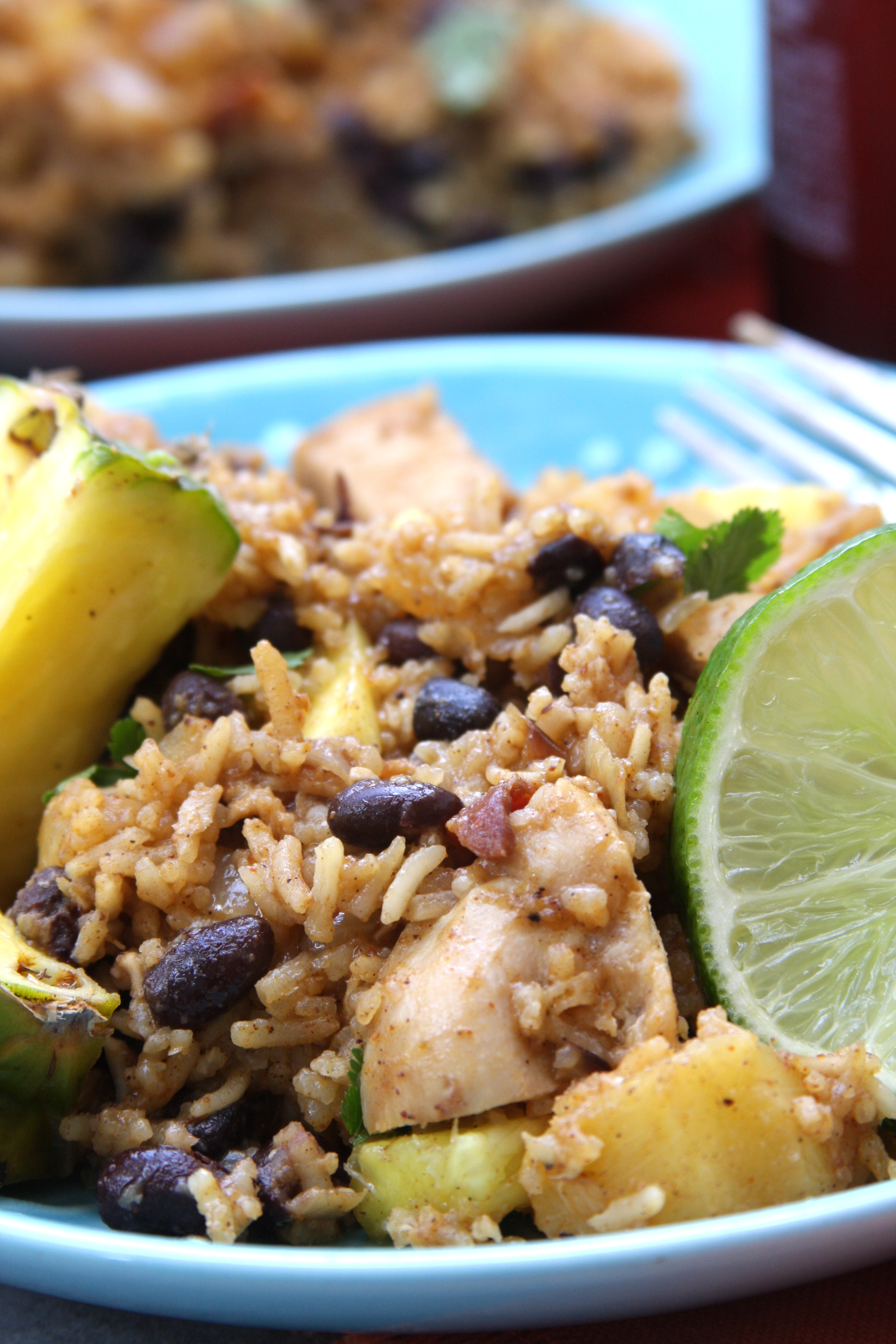This photograph captures a vibrant meal served on a blue ceramic plate, set against a reddish wooden table. The image is taken at a slight downward angle, offering a clear view of the beautifully plated food. The main dish appears to be a one-pot meal featuring a mix of brown rice and black beans. On the left side of the plate, there are several chunks of juicy, yellow pineapple, while on the right, a large, green lime wedge adds a touch of citrus flair, with its edge extending slightly out of the frame. Nestled among the grains and beans are small, white chunks of what seems to be pan-seared chicken, marked with a golden-brown sear.

Sprinkled across the dish are hints of fresh, green cilantro, contributing to the meal’s aesthetic and flavor complexity. The blue ceramic plate rests on a table that is slightly blurred, enhancing the focus on the meal. In the background, another similar blue plate with an identical dish is noticeable but out of focus, adding depth to the composition. A silver fork with its tines resting gently against the side of the plate completes this inviting culinary scene, suggesting a delightful mix of textures and flavors, possibly hinting at a Mexican-inspired dish.